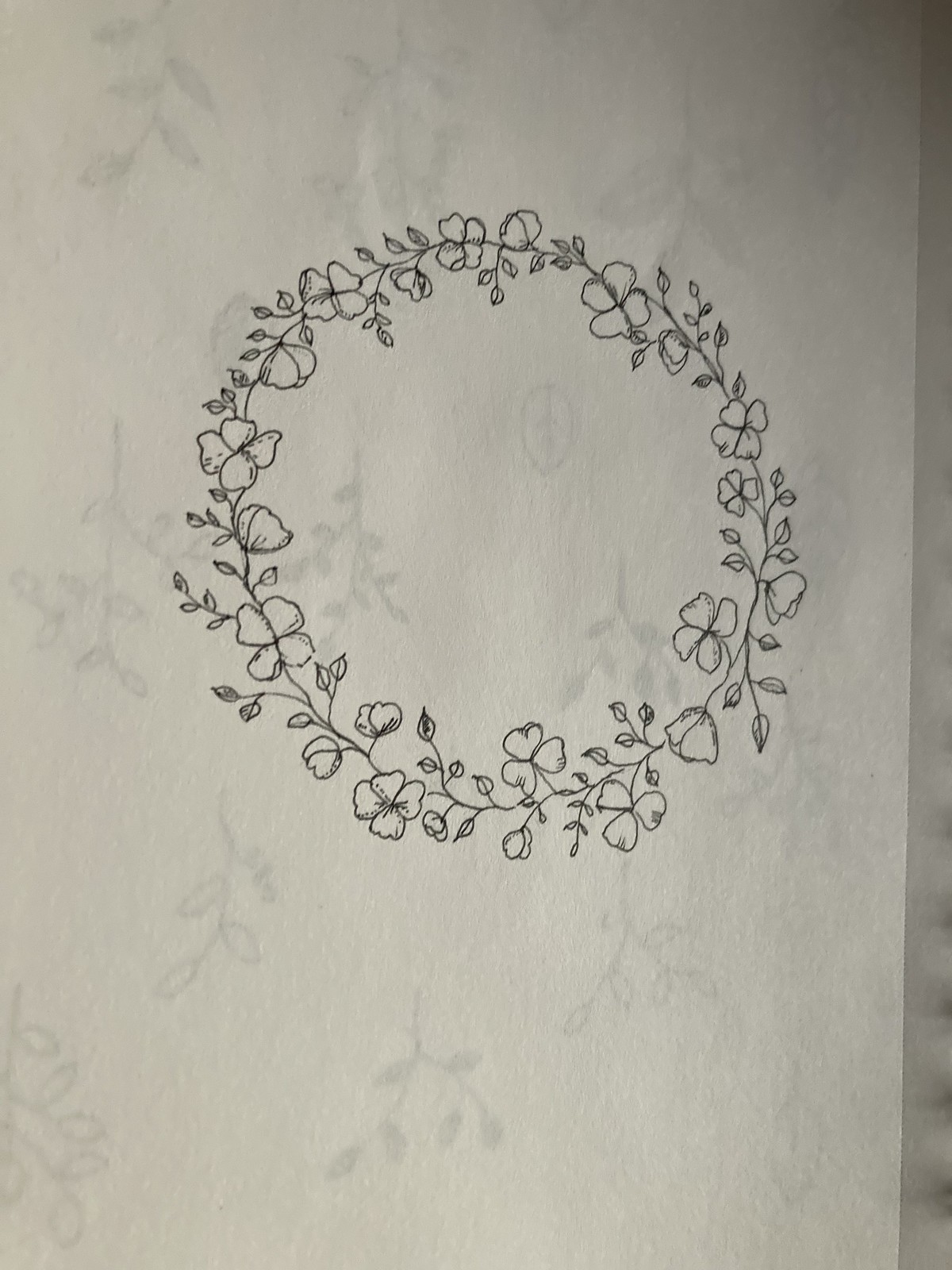This black-and-white image showcases an intricate drawing or pattern set against a white background. The design features a variety of flowers arranged in a circular formation, resembling a delicate wreath. The floral elements within the wreath exhibit a range of stages, from open blossoms to closed buds, along with accompanying leaves. The entire composition is rendered in thin, precise lines, imparting a hand-drawn quality that suggests it may have been created with a pen. The image is purely visual, containing no text, and emphasizes the subtle interplay of shapes and textures within the monochromatic palette.